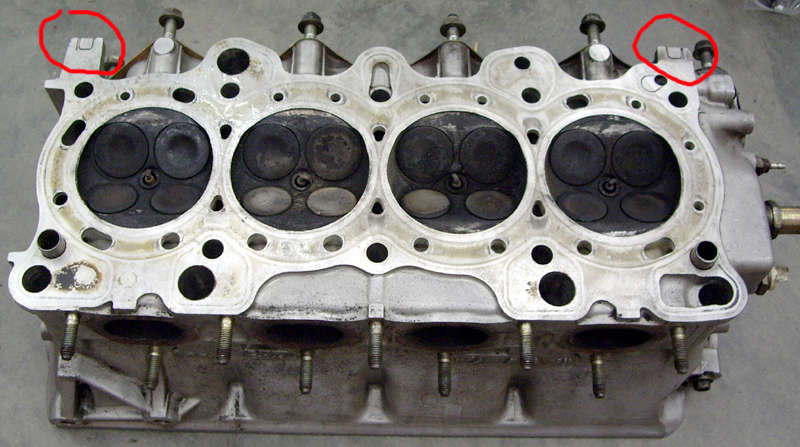This detailed photograph depicts a silver-colored engine block, possibly an automotive part, situated on a plain gray surface, likely concrete. The engine block, which is rectangular in shape, features four prominent circular openings aligned along its length. Each of these larger circles contains four smaller, lighter circles inside. There are numerous screws and holes peppered throughout the surface of the engine block, adding to its intricate, industrial appearance. The photograph has been edited to include orange circles around the top left and top right corners of the engine block, possibly to highlight specific sections for further attention. Additionally, four indentations with vertical metal objects can be observed at the bottom of the block. The image is wider than it is tall and lacks any discernible text or labels to identify the precise nature of the machinery.